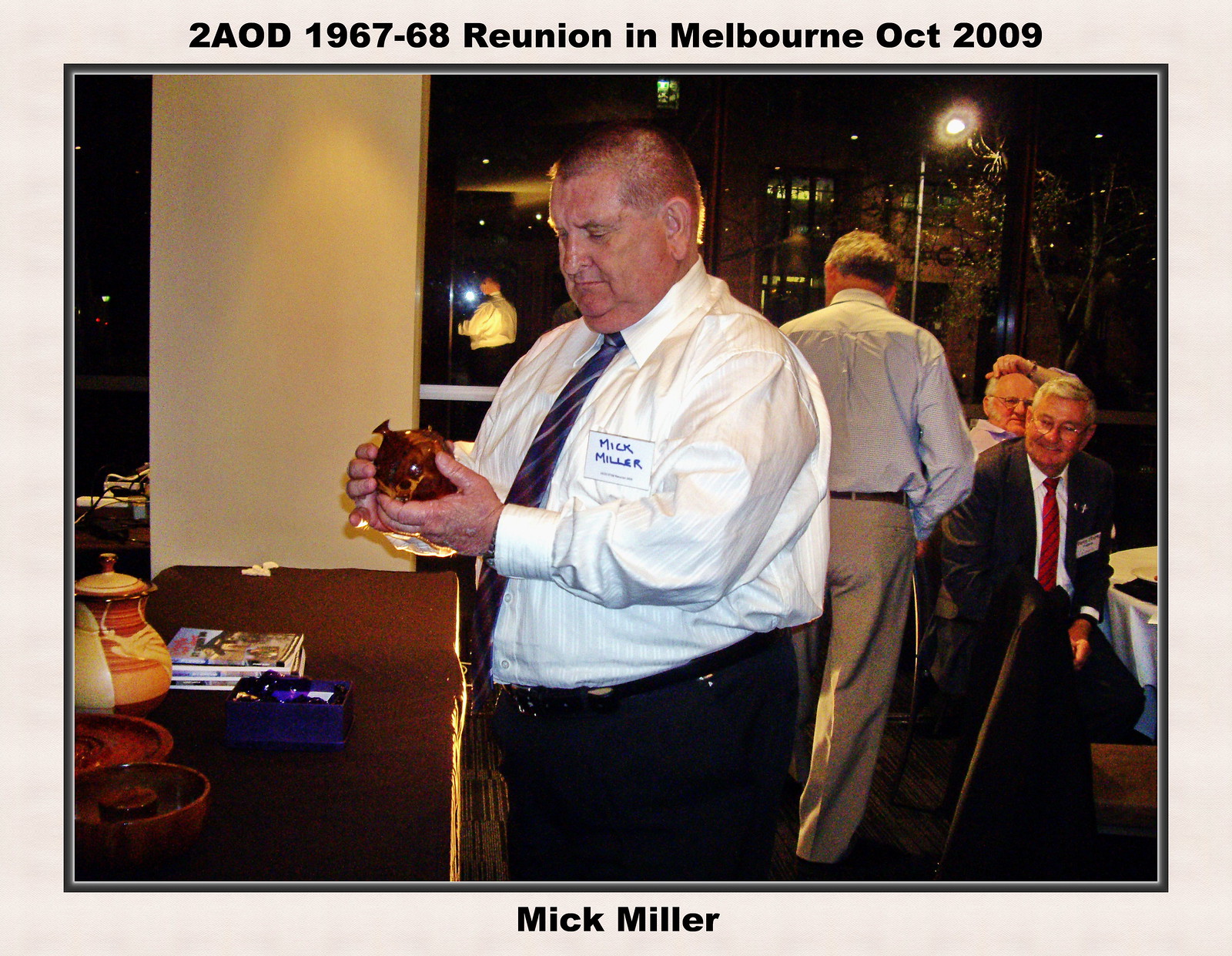The image captures a scene from the 2AOD 1967-68 Reunion in Melbourne, October 2009. At the center of the photograph stands an older, tall, and slightly overweight gentleman named Mick Miller, identifiable by his name tag. He is wearing a long-sleeved, white dress shirt, black pants with a black belt, and a dark tie adorned with white stripes. Mick Miller is holding a glass figurine in his hands, looking down at it intently. He is standing in front of a counter that displays an assortment of items including magazines, a blue box, and some glass and ceramic artifacts. In the background, three older men are visible—two are seated at a table in the midst of laughing, while the third is standing and appears to be walking towards the door. All of them are dressed in business attire. The setting appears to be a dimly-lit conference room or a restaurant, with large windows behind Mick reflecting his image and revealing a nighttime cityscape. The scene is framed with a white and thin black border, with text above the photograph reading "2AOD 1967-68 Reunion in Melbourne, October 2009" and the name "Mick Miller" inscribed at the bottom.